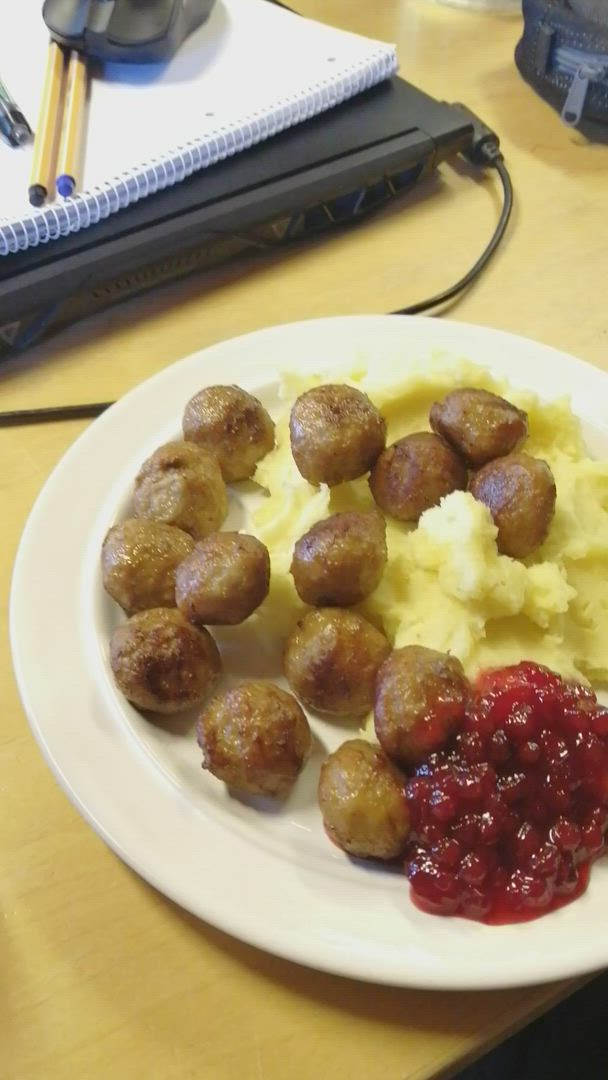This image captures a white circular plate centered on a light brown wooden tabletop. The plate features around 14 small, light brown meatballs, some of which rest atop a serving of yellow mashed potatoes on one side of the plate. Adjacent to the meatballs and mashed potatoes, at the bottom of the plate, is a dollop of reddish cranberry sauce with whole berries. Positioned behind the plate is a black laptop with a charger attached. A white spiral notebook lies on top of the laptop, accompanied by two yellow pens and a black mouse. In the upper right corner of the image, there is a small portion of a black bag with a gray zipper visible. The setup presents a contrast between the rustic meal and the modern, technology-filled workspace.